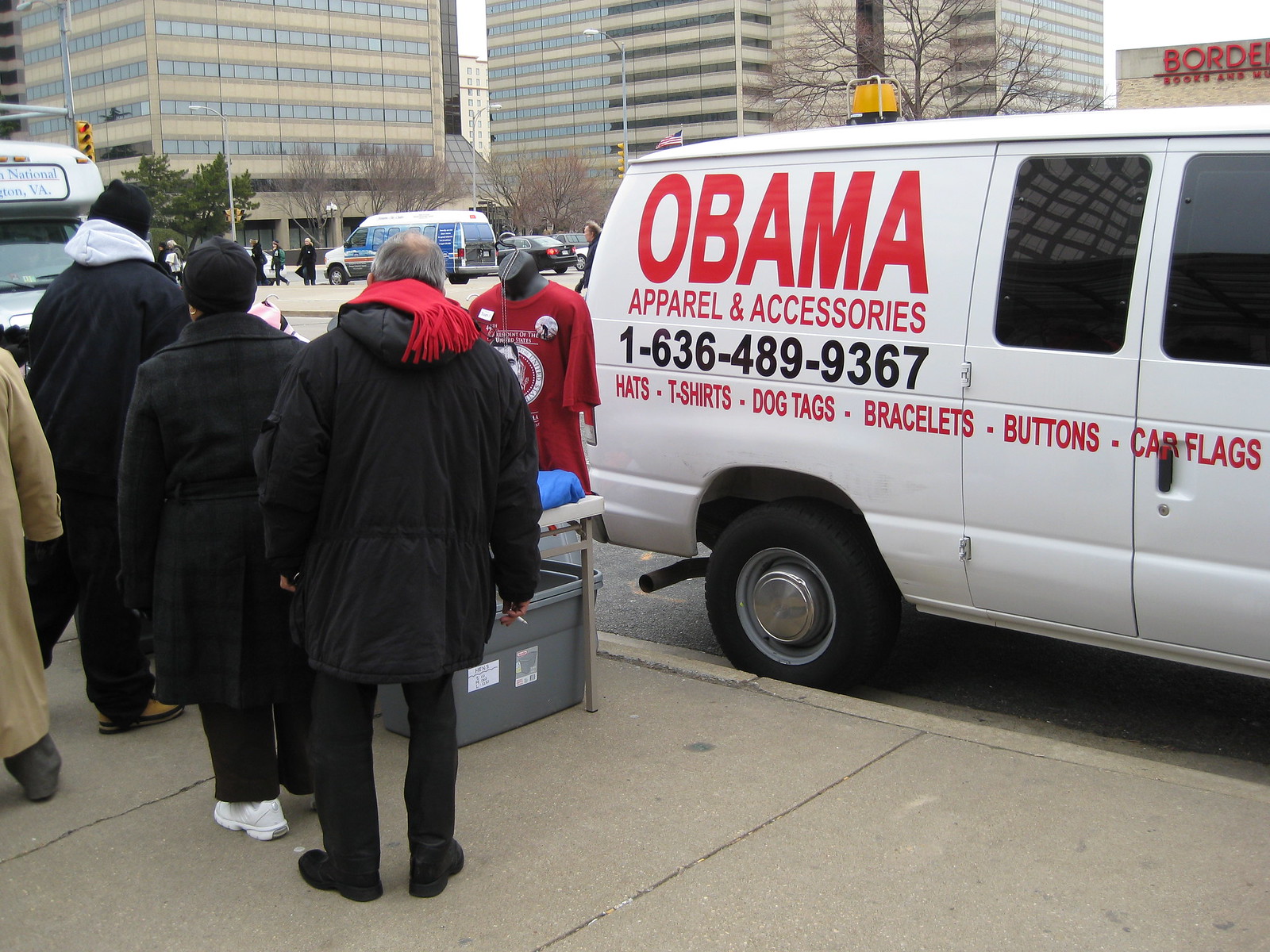In the midst of a bustling downtown cityscape, the photograph captures a sidewalk scene framed by towering high-rise office buildings in the background. Dominating the right side of the image is a white van adorned with bold red lettering that proclaims "Obama Apparel and Accessories." Beneath this header, smaller red text lists a selection of items: hats, t-shirts, dog tags, bracelets, buttons, and car flags, followed by a contact phone number in black. The van has an adjacent street vendor setup, featuring a table where merchandise, including a part of a mannequin dressed in a sweater, is displayed. Below the table, several totes are visible, likely containing additional stock.

On the left side of the image, several individuals—dressed in black coats and one in a tan coat partially cut off at the edge—are gathered around the display, seemingly interested in the merchandise. One person stands out with a red scarf, adding a splash of color to the otherwise muted winter attire, indicating a cold day despite the absence of snow. In the background, a city bus is visible on the far left, and between the tall buildings, a sign for a Borders bookstore can be spotted, suggesting the scene is set in a commercial downtown district. The overall scene portrays the enterprising spirit of a street vendor selling memorabilia and apparel celebrating Obama, set against the backdrop of a lively urban environment.